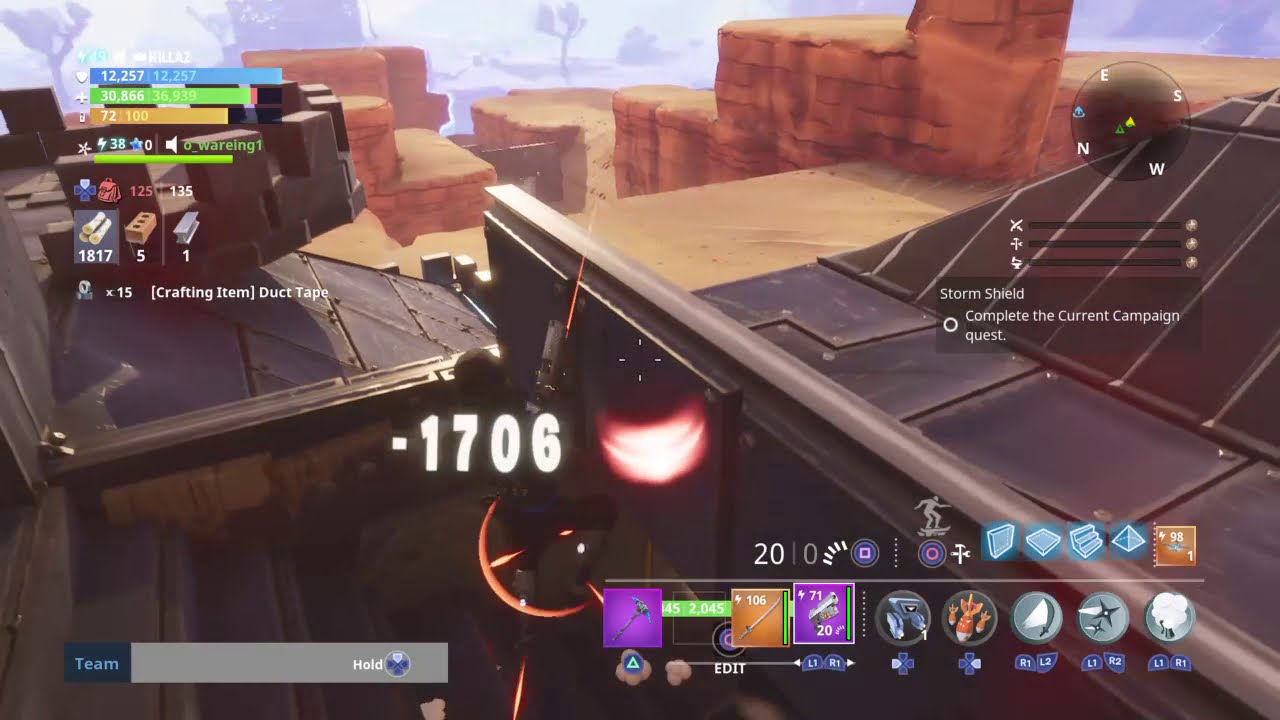This image is a detailed screenshot from a video game resembling Fortnite. The scene is set on the edge of a mountainous or desert area, with the player character standing atop a metal structure. The background features rock formations, brick walls, and a closing bubble on the horizon, indicating a shrinking game boundary. Dominating the middle of the screen is the large, white number "-1706," suggesting a negative score or status. Above this number is the text "Storm Shield," followed by "complete the current campaign quest." 

In the top left corner are the player's health and defense bars, displayed in green and blue, respectively, along with an inventory showing quantities of wood (branches), brick, and steel (I-beams). The bottom of the screen features the player's arsenal and crafting items. One notable crafting item is duct tape, with a quantity of "x15." Additional text at the bottom right provides indicators for available weapons and building modes. A compass in the right-hand corner aids navigation. The vibrant and dynamic interface gives a comprehensive view of the player's resources, progress, and challenges in the game, enhancing the immersive experience.